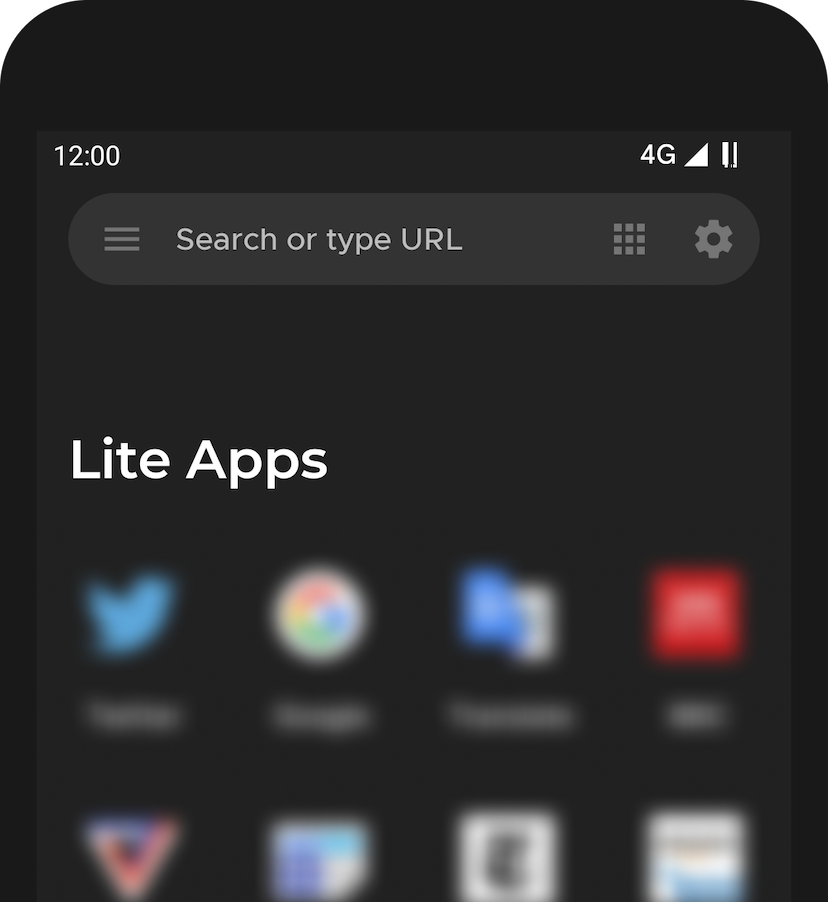This is a detailed close-up illustration of a black cell phone. The phone's screen is also black, with white text and icons displayed. At the top left corner, the time is shown as "12:00," while the top right corner displays "4G," along with icons for Wi-Fi signal strength and battery status. Below these indicators is a gray search bar, with the placeholder text "Search or type URL" in white. The search bar features a three-line menu icon on the left side and a grid icon followed by a settings cog icon on the right side.

Below the search bar, the text "Lite Apps" is prominently displayed in larger white lettering, spelling "L-I-T-E." Beneath this text are two rows of app icons, totaling eight in number. However, the icons are somewhat blurry, rendering most of them indistinguishable. The first app on the top row is identified as Twitter. The second app in this row features red, blue, yellow, and green in concentric circles. The rest of the apps display various color patterns, including combinations of white, blue, red, orange, dark blue, light blue, black, and green, but their specific identities remain unclear.